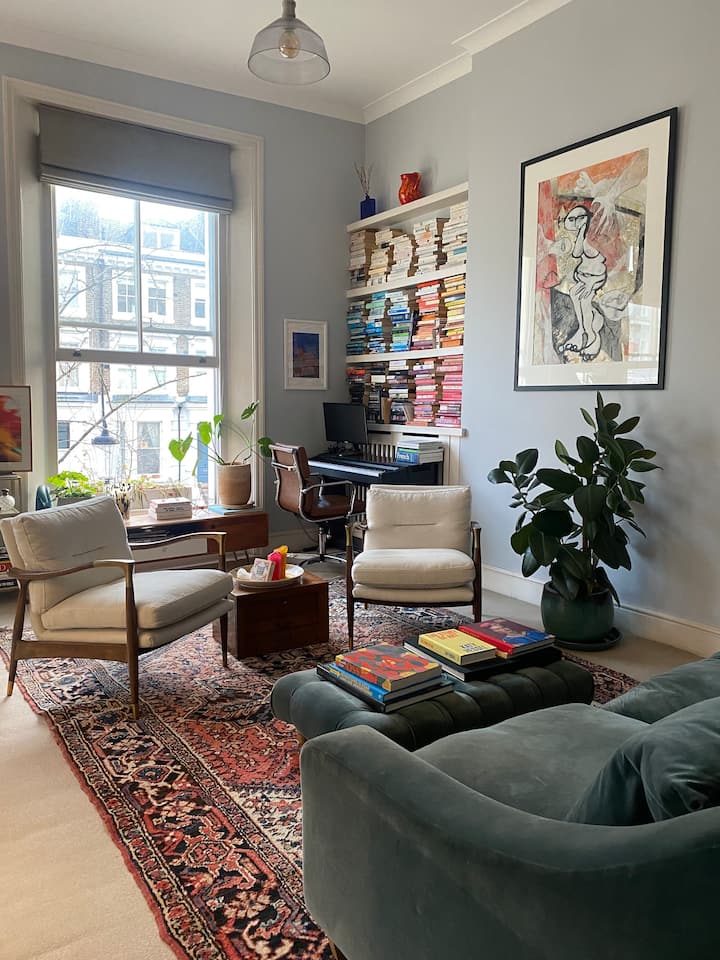The image depicts a cozy and well-decorated living room corner that exudes a comfortable and lived-in atmosphere. Dominating the floor is a rich, red oriental rug with intricate geometric designs and a wide border, covering most of the hardwood flooring. Centered in the room is a plush velvet blue armchair with a matching footrest, upon which several books are neatly stacked. Opposite this are two white armchairs with wooden frames, positioned to create a conversational area. Between the white chairs sits a small side table.

In the background, a desk with a brown, chrome-framed swivel chair and a computer monitor is set against the wall. Above and adjacent to the desk are shelves brimming with a variety of multicolored books. To the left of these chairs and closer to the back wall, a couple of feet tall potted plant thrives under a painting reminiscent of Picasso's style. The walls are painted in a slate gray color, enhancing the room's modern yet cozy vibe.

On the adjacent wall, a large floor-to-ceiling window with a rolled-up gray shade reveals an urban apartment landscape outside, possibly hinting at a New York-style setting. Small potted plants, a candle, and additional books adorn the desk area, emphasizing a blend of natural elements and a sense of personal space. Overall, the setting captures the essence of a multipurpose living room—serving as a conversation area, a library, and a workspace—bathed in a spectrum of colors from soft blues and greens to warm reds and khaki tones.